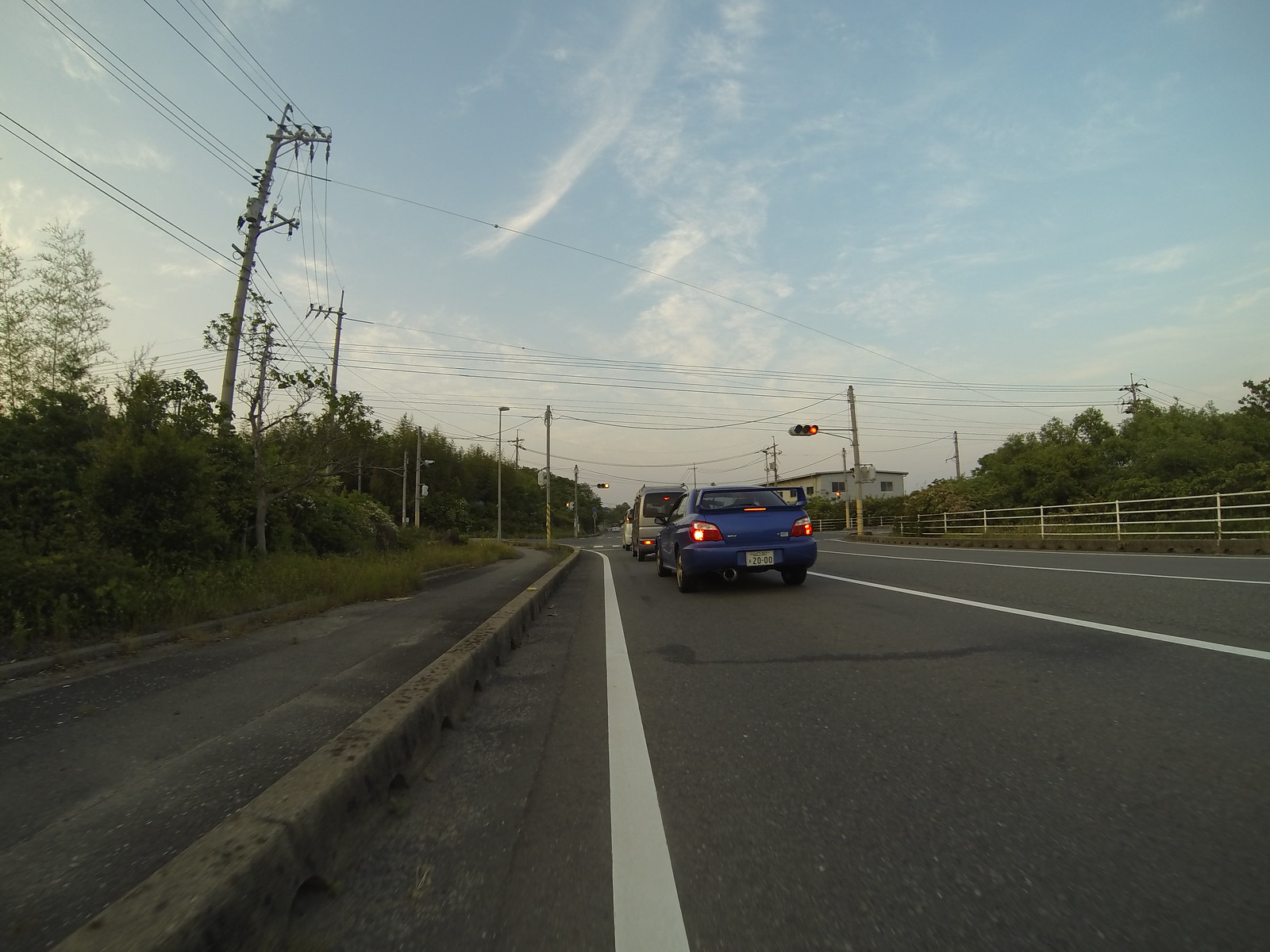The image depicts three cars stopped at a red light on a roadway in a country where drivers use the left side of the road, opposite to driving practices in the United States. The vehicles include a blue car in the back with its brake lights illuminated, a silver minivan also displaying its brake lights, and a red car further ahead without visible brake lights due to its distance. The traffic lights are mounted on poles at the side of the road, rather than hanging overhead as commonly seen in the US. The street is well-maintained and lined with numerous telephone poles, with wires running parallel to the road. On the far side of the street, a white picket fence stretches along the roadside. Above, a clear blue sky is dotted with wispy, white puffy clouds.